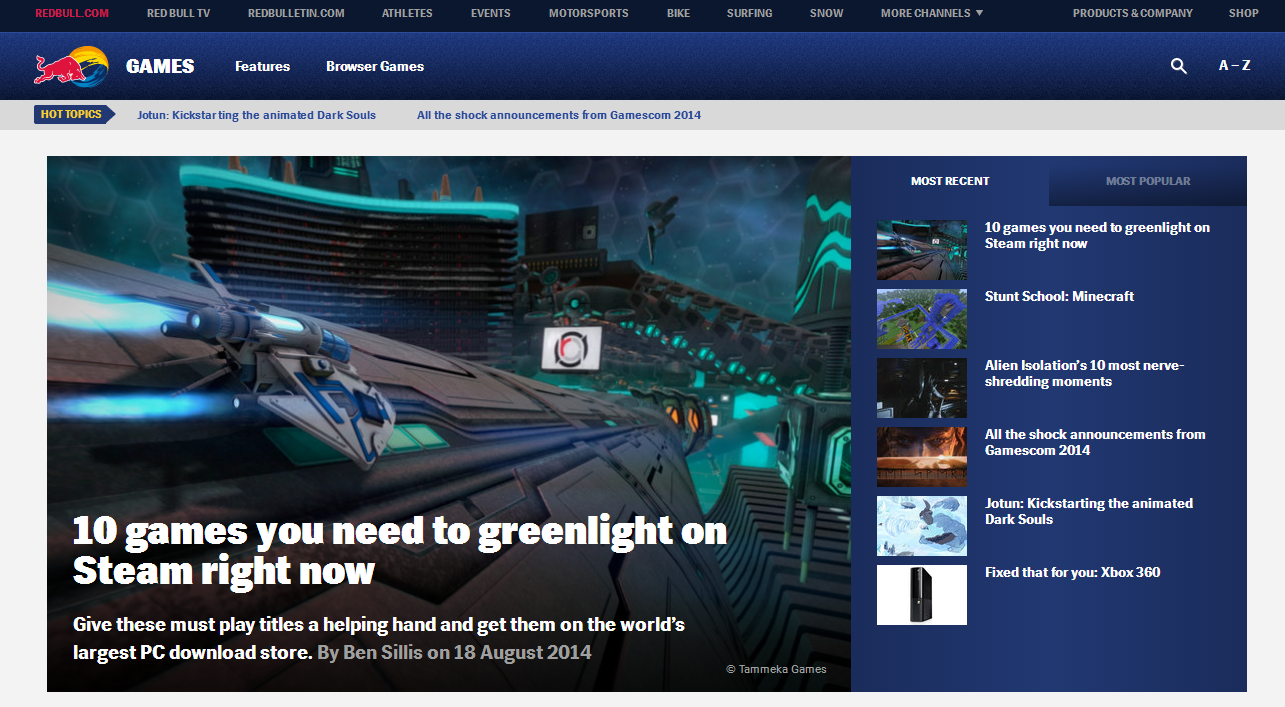The screenshot captures a section of a video game website featuring an article about science fiction racing games akin to F-Zero. The main article, titled "10 Games You Need to Green Light on Steam Right Now," written by Ben Sillis on August 18, 2014, encourages readers to support these must-play titles to get them available on the world's largest PC download store. 

To the right of this featured article are two tabs labeled "Most Recent" and "Most Popular," with the "Most Recent" tab currently selected. Under this tab, the article headlines are listed in order: "Stunt to School Minecraft," "Alien Isolation's 10 Most Nerve Shredding Moments," "All the Shock Announcements from Gamescom 2014," "Yoten, Kickstarting the Animated Dark Souls," and "Fix That For You: Xbox 360."

At the top of the page, the site's gaming focus is evident, with two highlighted "Hot Topics" articles being the ones previously mentioned. The website's header includes a logo and the word "Games," though the logo is too small to discern its exact design.